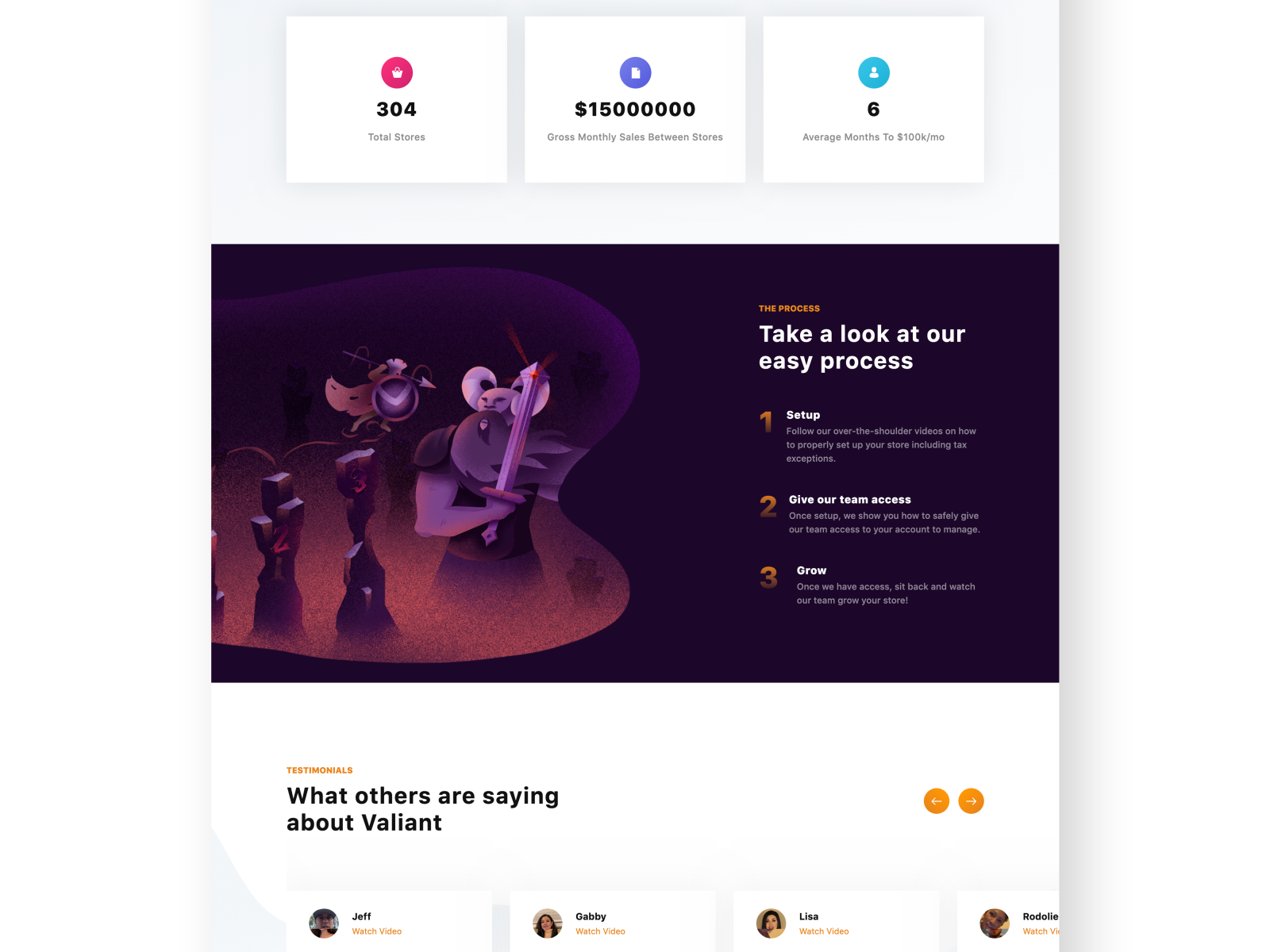A detailed web page interface with a dark gray background features distinct sections, each set within white squares containing various elements:

- **Top Section:**
  - A white square with a central red circle.
  - Below it, a white shopping bag icon.
  - Text reading "304" in bold black, with "Total Stores" in gray below.

- **Second Section:**
  - Another white square encases a purple circle holding a white sheet of paper with a dollar symbol inscribed. 
  - Text stating "$1,500,000" in bold black, followed by "Gross Monthly Sale Between Stores" in gray.

- **Third Section:**
  - A dark blue square containing a white silhouette of a person.
  - Text reading "6" in bold black, with "Average Months to 100K/mo" in gray beneath.

Following these sections is an animated figure resembling a Viking warrior with white horns on his helmet. He stands next to two stone statues, one featuring a "2" in red, the other a "3," both brown. The Viking character wears brown leather armor and a blue kilt, enclosed in a bubble that transitions from brown at the bottom to purple at the top. This segment rests on a dark blue background. 

To the right, orange text spells out "The Process," accompanied by bold white text stating, "Take a look at our easy process." Below are three distinct steps:

- **Step 1:** 
  - Orange number "1" with bold white text "Set Up."
  - Gray text: "All our over-the-shoulder videos on how to properly set up your store, including tax encryptions."

- **Step 2:**
  - Orange number "2" with bold white text "Give Our Team Access."
  - Gray text: "Once set up, we show you how to safely give our team access to your account to manage."

- **Step 3:**
  - Orange number "3" with bold white text "Grow."
  - Gray text: "Once we have access, sit back and watch our team grow your store."

At the bottom of the page, an orange heading reads "Testimonials," with bold black text stating "What Others Are Saying About Valiant."

Below are profile sections of various staff members, each within white rectangles, with profile pictures, bold black names, and orange "Watch Video" buttons beneath. The staff includes:

- **Jeff:** An olive-skinned individual wearing a black shirt and hat.
- **Gabby:** A female with shoulder-length brown hair, a black shirt, and hand resting against her face.
- **Lisa:** A person holding a brown and tan book, sporting short black hair and pink/red lipstick.
- **Rodolie:** An olive-skinned woman turning to the side, donned in a blue shirt.